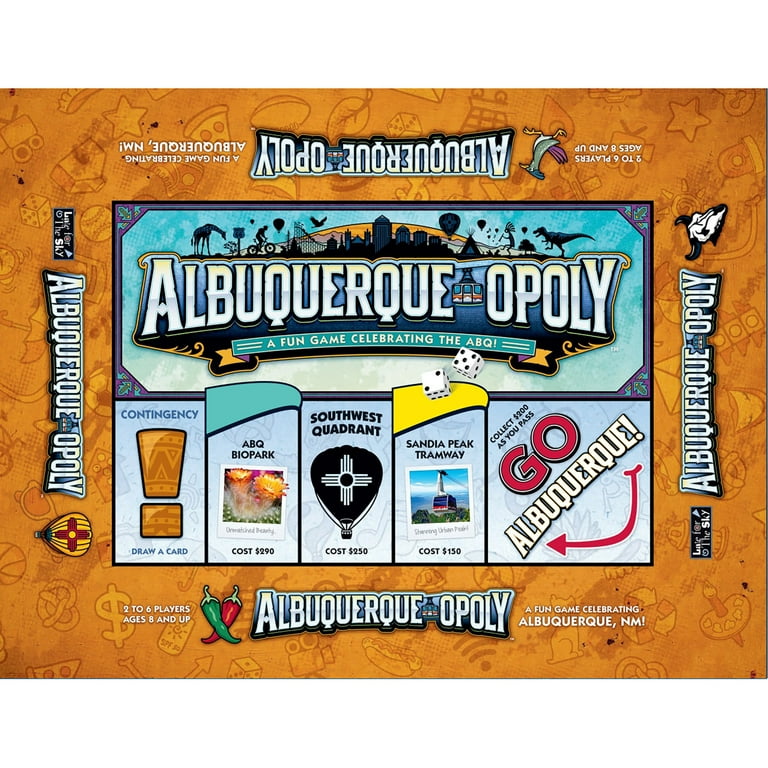The image depicts the box of a themed board game called "Albuquerque-Opoly," which is styled similarly to Monopoly. The title "Albuquerque-Opoly" is prominently displayed in large white letters at the bottom of the box, accompanied by a red and green jalapeño to the left. The tagline "A fun game celebrating Albuquerque, New Mexico" is also present. The game is designed for 2 to 6 players, ages 8 and up. 

The background of the box features a brown, tan-toned surface adorned with various illustrations such as a star, pretzels, money signs, and pieces of pizza. The sides of the box repeat the "Albuquerque-Opoly" title, with different images angled at various orientations, including a cow skull, a hot air balloon, and a bird with purple tail feathers.

The detailed game board includes various spaces with local Albuquerque landmarks and costs, such as "Contingency," "ABQ Biopark" costing $290, "Southwest Quadrant" costing $250, and "Sandia Peak Tramway" costing $150. It also features the classic Monopoly starting point, "Go," with the instruction to "Collect $200 as you pass." Dice are also included in the game setup, indicating it is a board game that uses dice for movement, much like the traditional Monopoly.